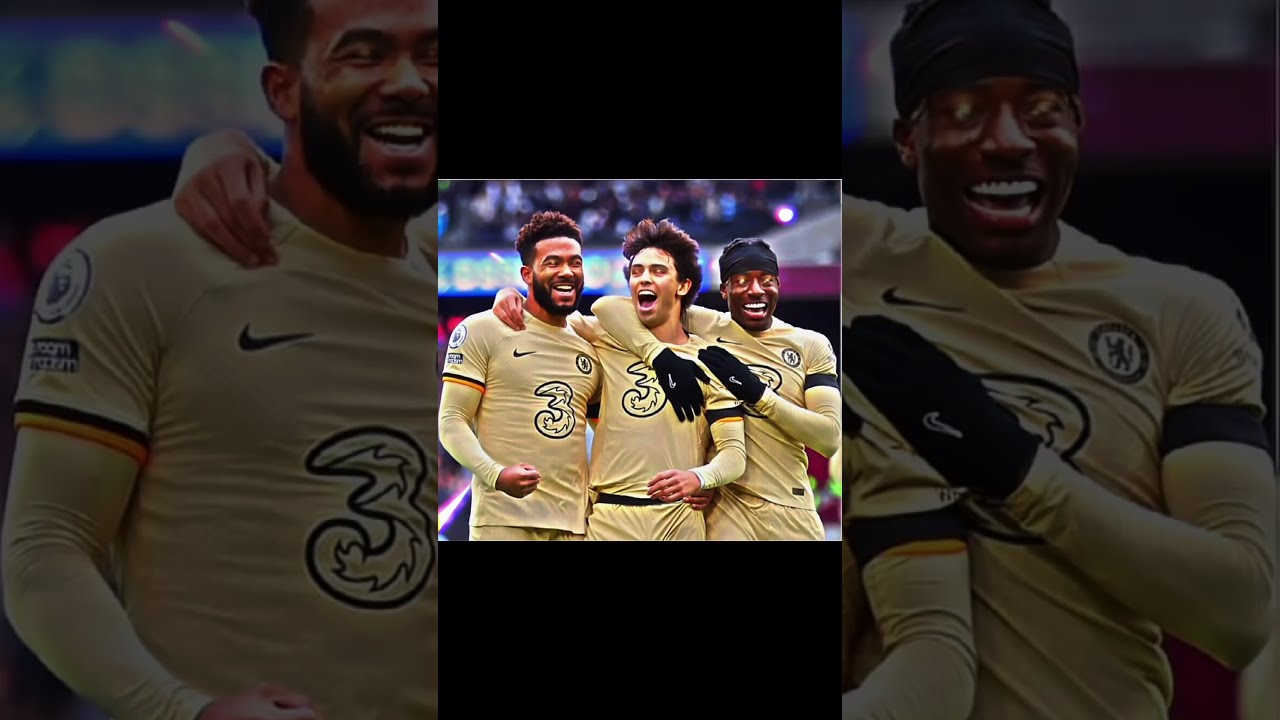The image is a postcard-style collage divided into three rectangular sections, each dimmed to about 50% lighting. At the center, where the focus lies, a vibrant, letterboxed image shows three exuberant young men dressed in matching mustard yellow jerseys emblazoned with the number three in a doodle-style font. The men, all with medium-length hair, have their arms draped around each other, exuding joy and camaraderie. The man on the left, an African American, has darker brown skin and sports a blue headband. In the middle, a Caucasian man with lighter skin stands with a big grin. On the right, another African American man with even darker skin is distinguishable by his black gloves. Their shorts or pants match the white sleeves of their jerseys. Each top prominently features a black Nike Swoosh logo on the chest, indicating probable team sponsorship. The left and right sections of the collage provide close-ups of the leftmost and rightmost men, highlighting their cheerful expressions, while the central image brings the team spirit to life.